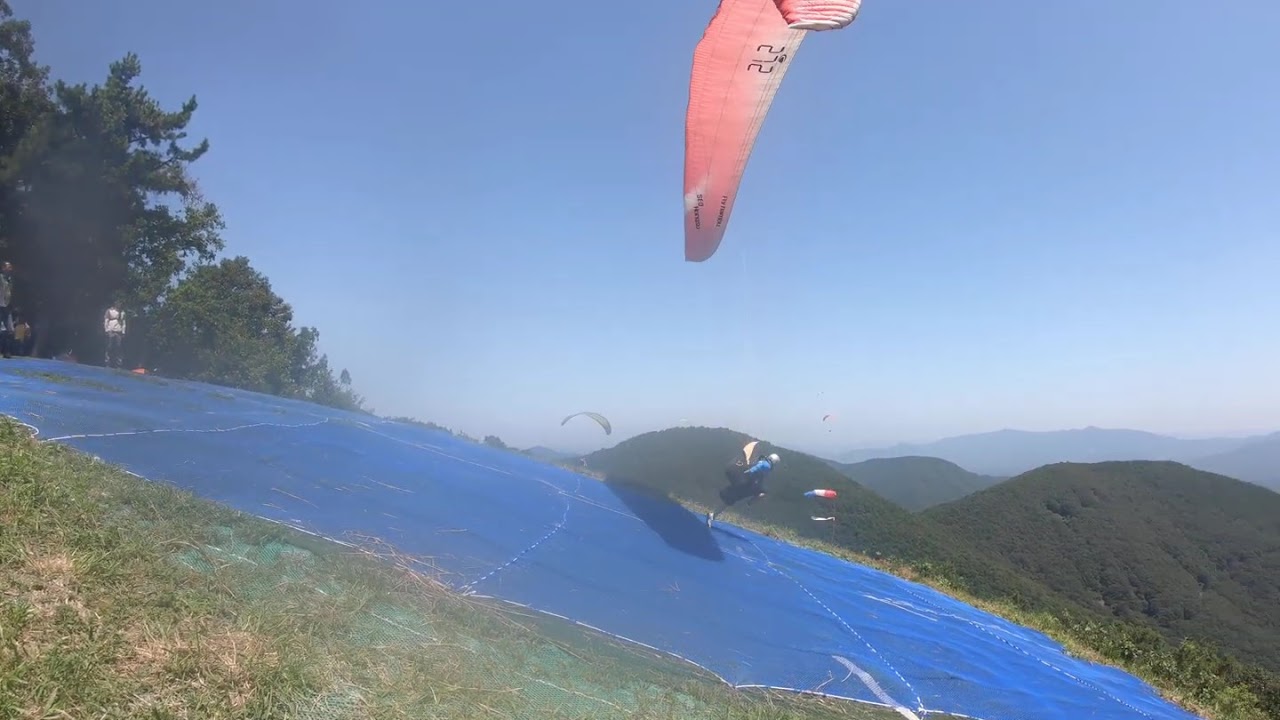The image depicts a vibrant outdoor paragliding scene on a sunny day. The lower right section of the image showcases a hillside covered in lush green trees. In the foreground, on the slope of the hill, a large blue tarp serves as a launch pad for paragliders. A person wearing a blue top and a whitish helmet is seen paragliding, their pinkish-coral banana-shaped parachute just a foot off the ground as they take off from the launch pad.

In the upper left, there's a grouping of trees where a person in a white shirt and another indistinguishable individual stand, observing the activity. Additionally, a red, white, and blue windsock indicates the wind direction, favoring the uphill area. Beyond this launch area, the landscape unfolds into beautiful, rolling green hills and further distant mountains that appear bluish due to the atmospheric perspective.

The clear blue sky makes for ideal flying conditions, and you can spot two more paragliders in the background: one about 100 feet away, and another smaller and more distant at around 200 feet away. The paragliding and picturesque environment create a serene yet exhilarating scene.